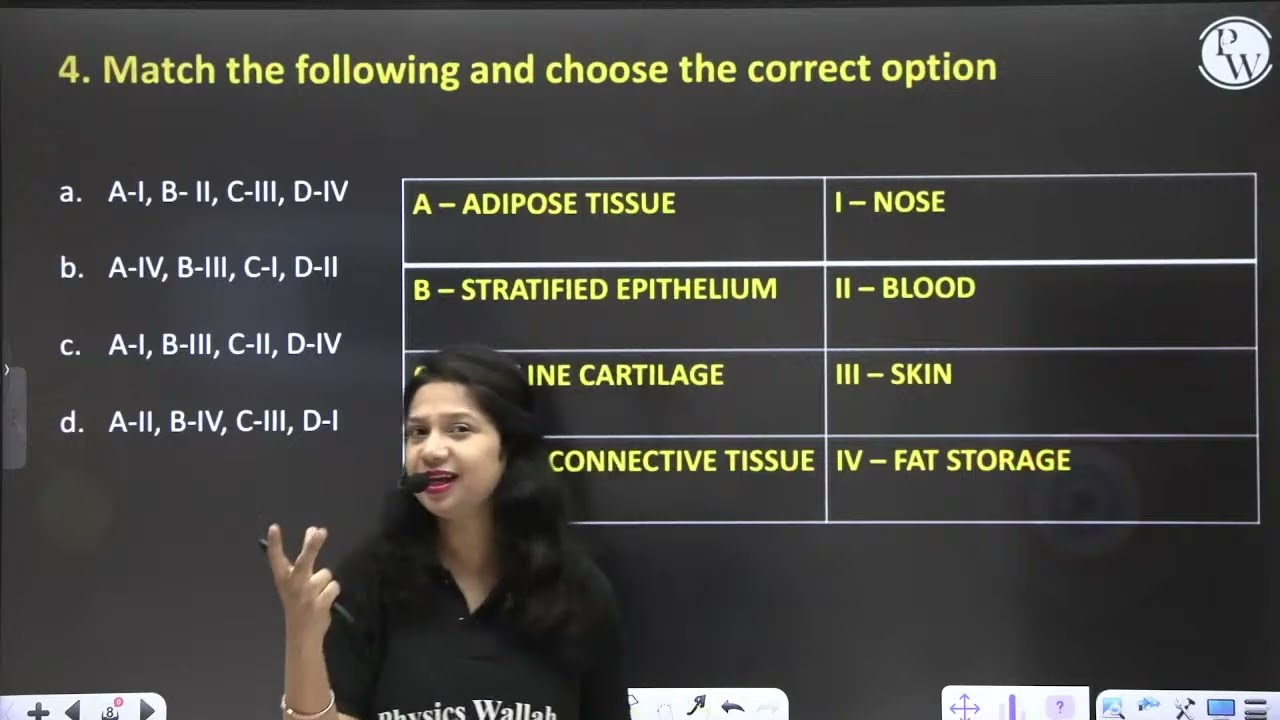A woman with long black hair, wearing a black shirt and red lipstick, stands in front of a gray blackboard or slide. She has a headset microphone near her mouth and holds a marker or pen in one hand, with three fingers extended. The blackboard features a title in yellow at the top that reads "4. Match the following and choose the correct option." Below this title on the left, the letters A, B, C, and D are listed with corresponding phrases starting with A, such as "A - 1, B - 2, C - 3, D - 4" and "A - 4, B - 3, C - 1, D - 2," with the numbers in Roman numerals. On the right side of the blackboard is a table with four rows and two columns. The left column labels include terms like "A Adipose Tissue," while the right column pairs them with "1 - Nose" and other health-related terms such as "blood, skin, and fat storage." Additionally, in the upper right corner of the board, there's a circular logo with the letters "PW" in white and gray. The woman appears to be conducting a lesson or stream, possibly discussing topics related to health.